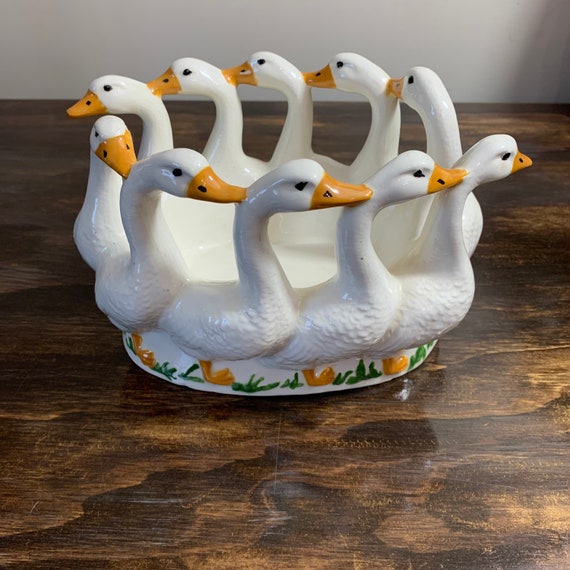On a finely polished, wavy-grained wooden table set against a white wall with a slight shadow, sits an intriguing decorative ceramic bowl. The bowl features a ring of 10 interconnected white geese with orange bills, each goose's beak touching the back of the neck of the one in front, creating a continuous circle. The geese are positioned in a counter-clockwise motion, with alternating directions for their heads—geese in front looking right and those in back looking left. The bowl is quite shallow and embellished with painted green grass at the base, adding to its ornate design. The ceramic piece, likely more decorative than functional, shows a meticulous attention to detail, such as the single orange leg visible for each goose and distinct black eyes.